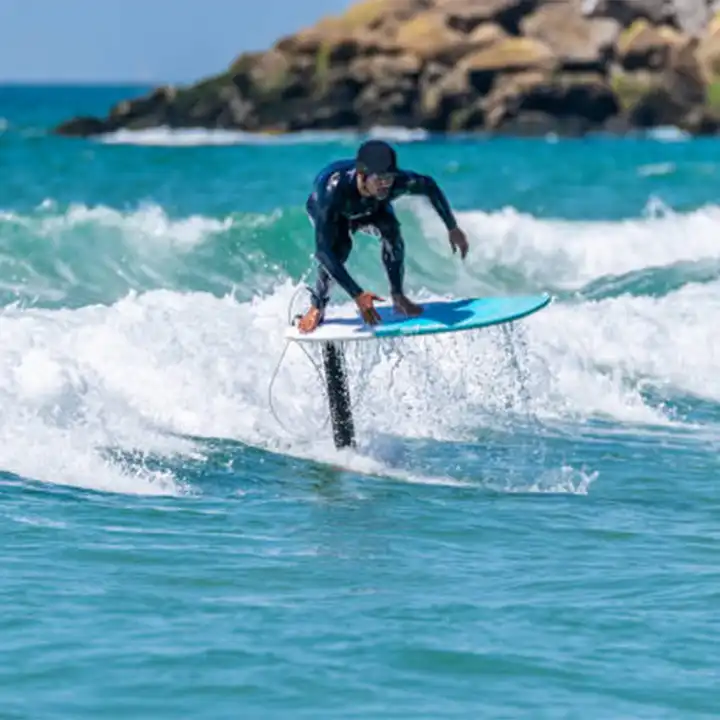This vibrant and somewhat blurry daylight photograph captures a thrilling moment of a man riding a hydrofoil surfboard over the ocean's surface, with the noticeable background of a rocky, mountainous landmass jutting out over the water on the right. The surfer, positioned prominently in the center, is crouched low on a teal and white surfboard that mimics the swirling blues and aquas of the sea. Notably, the surfboard is elevated a few feet above the foamy white wave, thanks to a black hydrofoil column attached to its back, creating an illusion of flying over the water. His dark blue wetsuit, paired with a matching cap and dark goggles, adds to the dynamic, almost futuristic scene. A safety link connecting his ankle to the board is also visible. Despite the image's overall lack of sharpness and definition, it conveys the energy and beauty of the sport against the stunning oceanic backdrop.